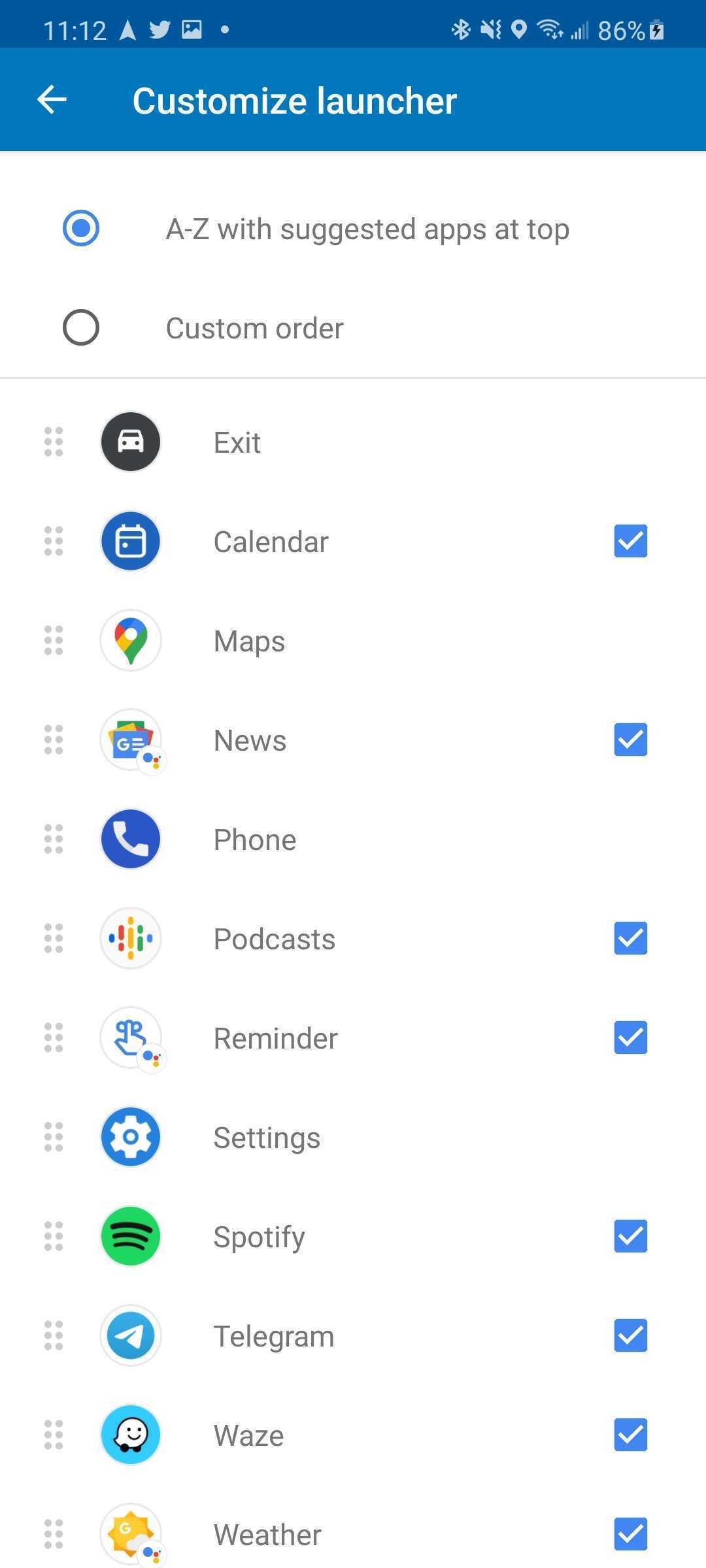A detailed caption for the screenshot provided:

"This screenshot, taken from a smartphone, clearly showcases various interface details indicating it is a phone. At the top left of the screen, the current time is displayed as '11:12,' accompanied by several icons including a Twitter icon (depicting a bird) and a picture icon, which suggests a screenshot notification. On the top right, the battery status shows as 86% with a black lightning bolt icon indicating that the phone is currently charging.

The main content of the screenshot pertains to a page titled "Customize Launcher," set against a blue background with a left-pointing back arrow at the top left corner. Directly below this heading, a button labeled 'A to Z with Suggested Apps' is highlighted, indicating it is selected. Adjacent to this, another button labeled 'Custom Order' remains unselected.

Below these options is a list of apps displayed in a specific order. The first app listed is 'Exit,' followed by 'Calendar.' Several apps have a blue checkmark beside them, indicating selection. These apps include Calendar, News, Podcasts, Reminders, Spotify, Telegram, Waze, and Weather."